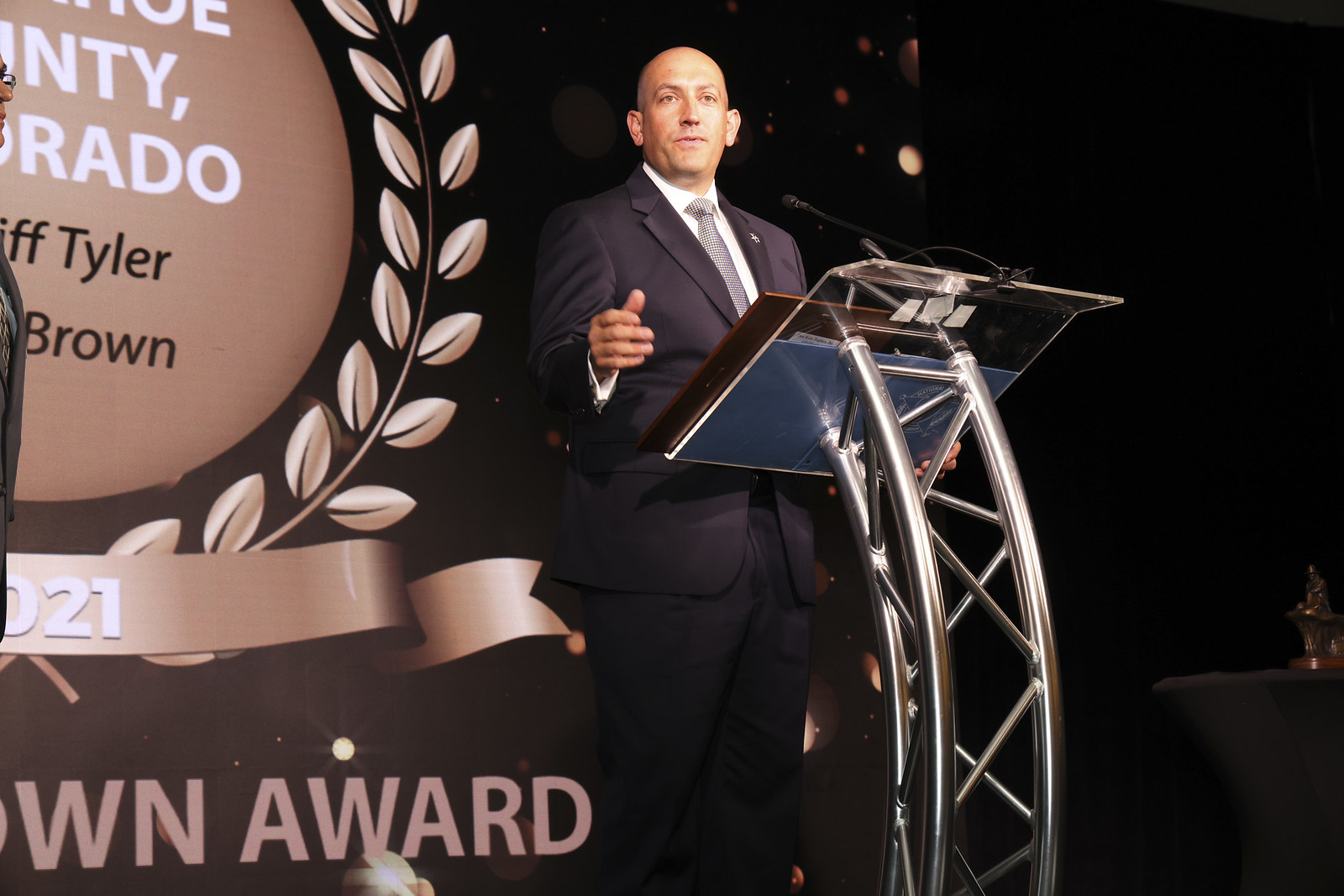In the image, a bald man dressed in a blue suit with a white buttoned-down shirt and a blue tie stands behind a small, clear glass podium with a metal base. His right hand is bent at the elbow, raised to chest height with his fingers slightly curved, as if gesturing while speaking. He's in mid-speech, facing the audience. The podium also features a microphone attached to it. Behind him, a dimly lit interior forms the backdrop, drawing attention to the brightly lit stage. A large banner, adorned with wheat laurels and emblazoned with partial text and a ribbon that possibly reads "2021," hangs to his left. Some visible letters on the banner include “NTY,” “RADO,” “IFF,” “Tyler,” and “WN award,” though parts of the words are cut off. In the bottom right corner of the image, a trophy can be seen lying in the darkness, adding to the ambiance of what appears to be an award ceremony. The man's facial expression is neutral, focused on delivering his speech to the audience.